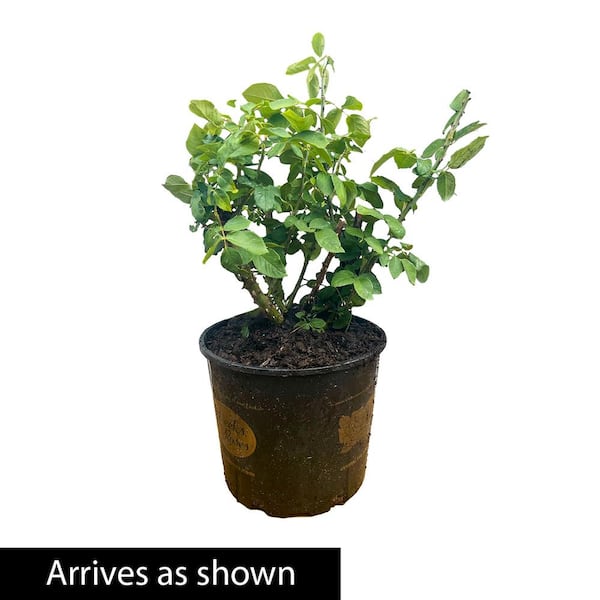This is a detailed photograph of a potted plant, showcasing what appears to be a young shrub with thorny, slender stalks and numerous small, waxy green leaves. The plant sits in a rich, dark brown plastic pot, which has a tan logo and text that is hard to read. The soil and mulch around the plant appear moist, giving the pot a well-watered look. The pot is large enough to suggest it can be used outdoors, although it could also be placed indoors with an additional protective base to prevent water damage. The lower left-hand corner of the image features a white text in a black rectangular box that reads "arrives as shown," indicating this is a promotional photograph, likely for an advertisement or a catalog, depicting the product's appearance upon delivery.